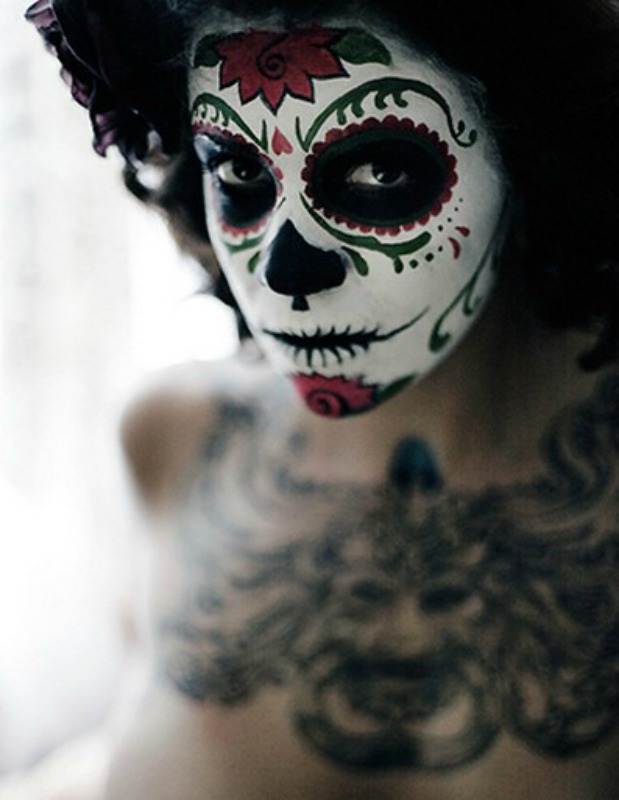This photograph features a woman elaborately dressed up for Dia de los Muertos. Her face is painted to resemble a skull, with a bright white base. Black surrounds her eye sockets, nose tip, and lips, which are adorned with black-and-white stripes mimicking skeletal teeth. Red roses embellish her chin and forehead, accentuated by green vines and stylized eyebrows that frame her striking eyes, further highlighted by additional red petals. Her dark hair contrasts with her vibrant face paint. The focus is on her detailed facial art, though a large, blurred tattoo covering her chest and torso is partially visible, depicting a tribal, demonic face or mask. She may also be wearing a hat, adding to her festive Dia de los Muertos attire.